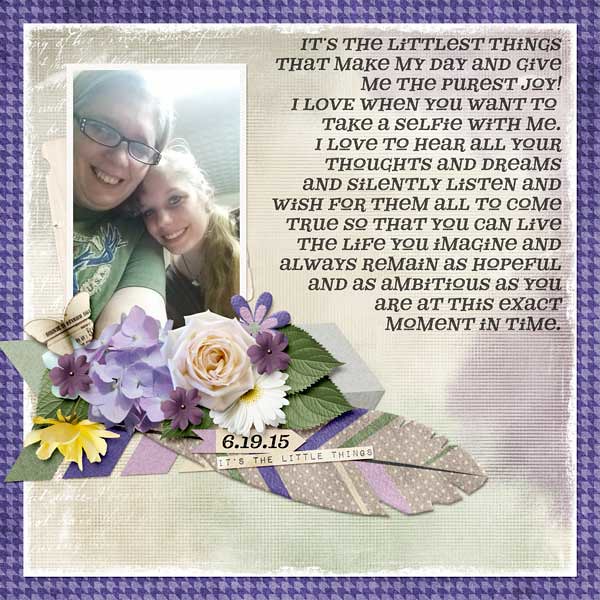This image appears to be a scrapbooking card with a blue and black decorative frame. The card is square with a light gray background and features a picture in the upper left-hand corner of a mother and her daughter, who looks to be in her 30s. The mother has short gray hair, glasses, and is wearing a green shirt, while the daughter has long blonde hair. The daughter rests her head on her mother's shoulder, and both are smiling at the camera, seemingly taking a selfie. Below their picture, there is an arrangement of purple, white, and yellow flowers, along with the date 6-19-15 and the phrase "it's the little things." The right side of the card contains 15 lines of printed text in black letters, which reads: "It's the littlest things that make my day and give me the purest joy. I love when you want to take a selfie with me. I love to hear all your thoughts and dreams and silently listen and wish for them all to come true so that you can live the life you imagine and always remain as hopeful and as ambitious as you are at this exact moment in time." There are also artistic paper cutouts of feathers below the flowers.